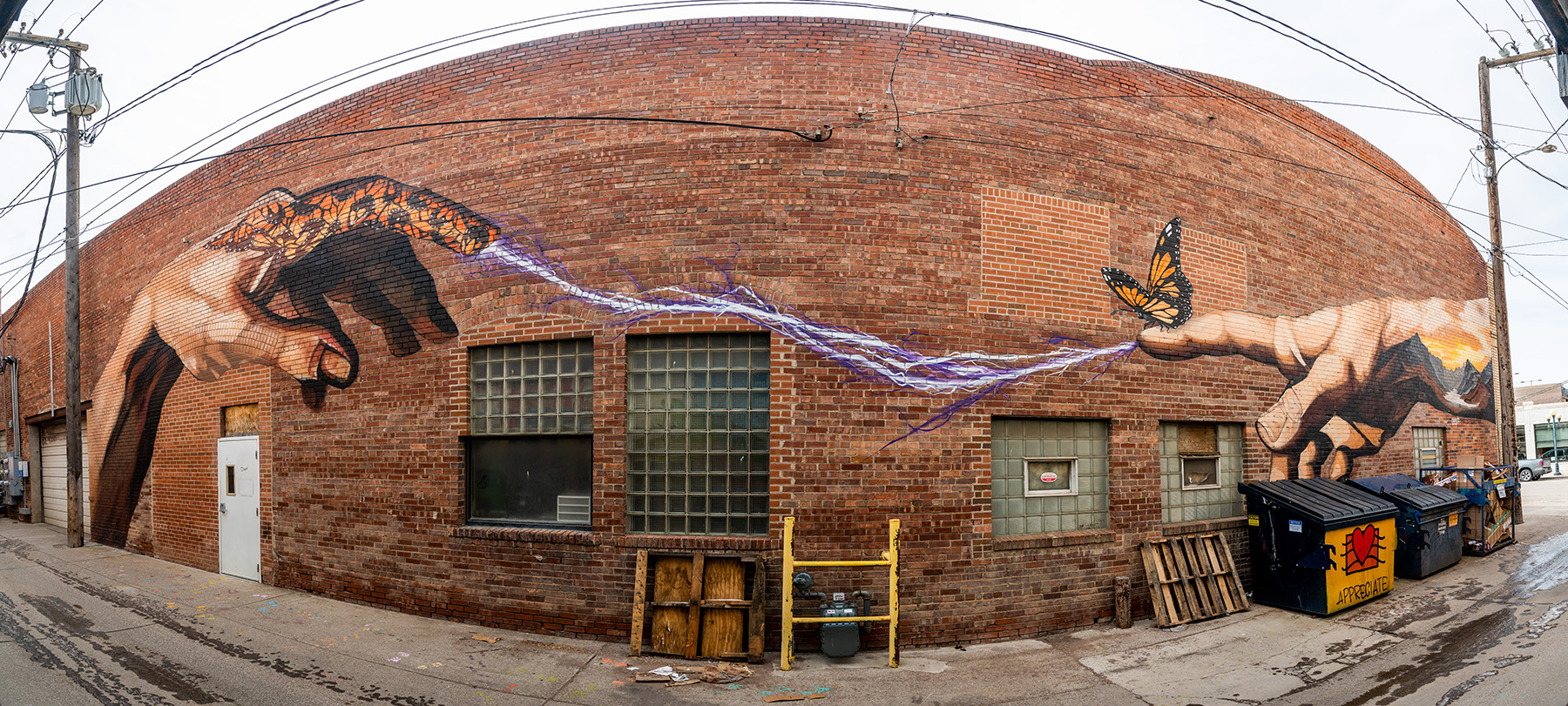The photograph captures a vibrant mural painted on the side of a red brick building, taken with a panoramic effect that curves the otherwise straight architecture. The scene is set outdoors under a clear sky, featuring brown electrical poles with numerous wires and an unlit streetlamp in the top right corner. The building's red brick exterior includes several windows, a white garage door on the left, and various pieces of scrap wood and black dumpsters are scattered in the alleyway in front. Dominating the mural are two oversized hands — a left hand on the left and a right hand on the right — with their index fingers extended towards each other. The left index finger is uniquely adorned in a monarch butterfly pattern, and a monarch butterfly perches delicately on the right hand's index finger. A bolt of purplish lightning arcs dramatically between the fingertips, evoking the iconic imagery of an electrical connection.